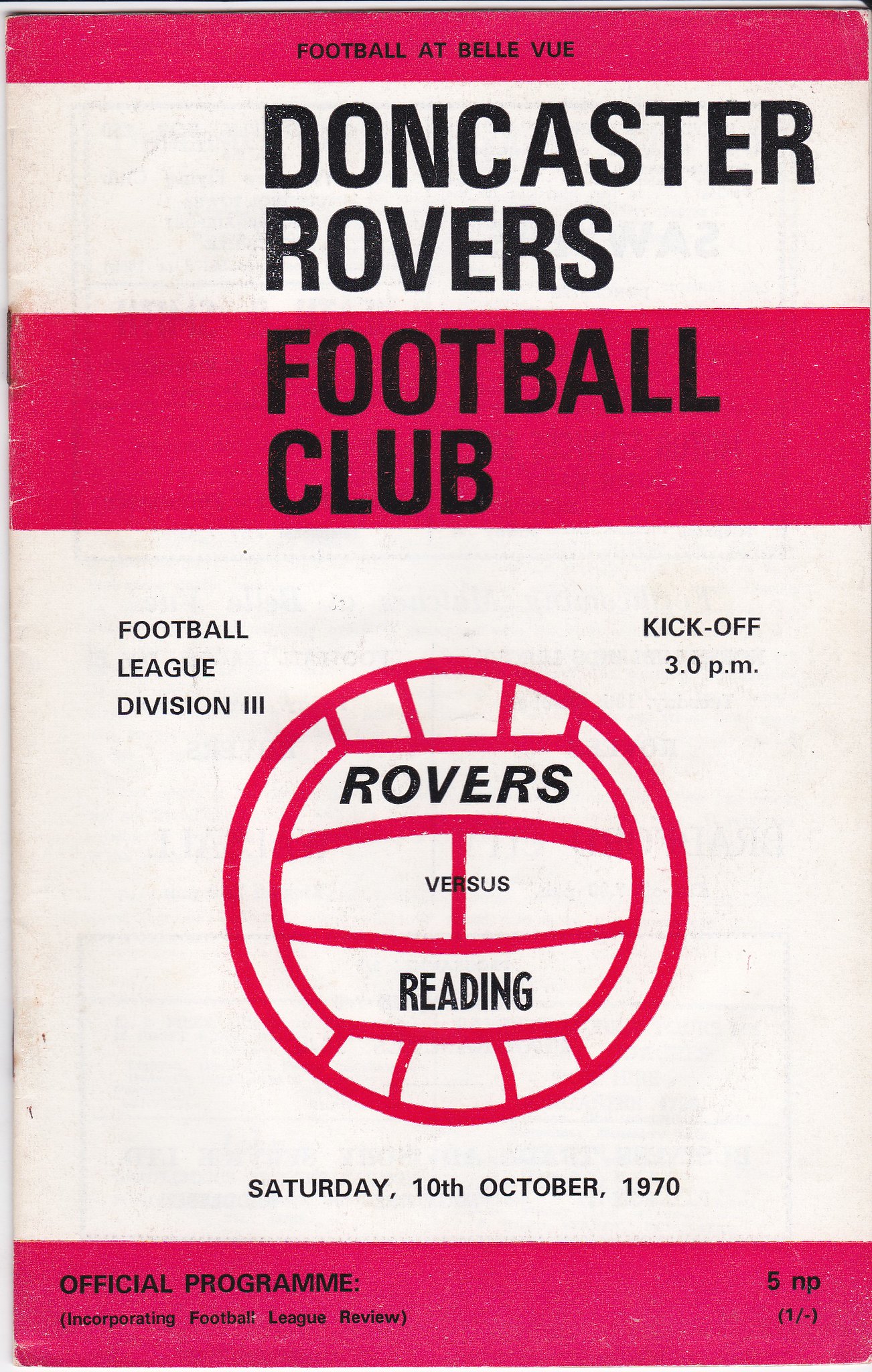The image features a vintage official program from 1970 for the Doncaster Rovers Football Club, prominently designed in white and shades of pink. At the top, the text reads "Football at Bellevue," followed by "Doncaster Rovers Football Club" in large, bold letters. Below this, it states "Football League Division 3 Kickoff 3 p.m. Saturday, 10th October 1970," indicating the match details, "Rovers versus Reading." The centerpiece of the poster is a stylized illustration of a soccer ball set against a large white background, framed by alternating hot pink and white bands. The bottom pink bar reads "This is the official program incorporating Football League Review," and the price, "5NP," is noted to the right. The dominant colors of the design are red, white, and pink, giving the program a vibrant and eye-catching appearance.